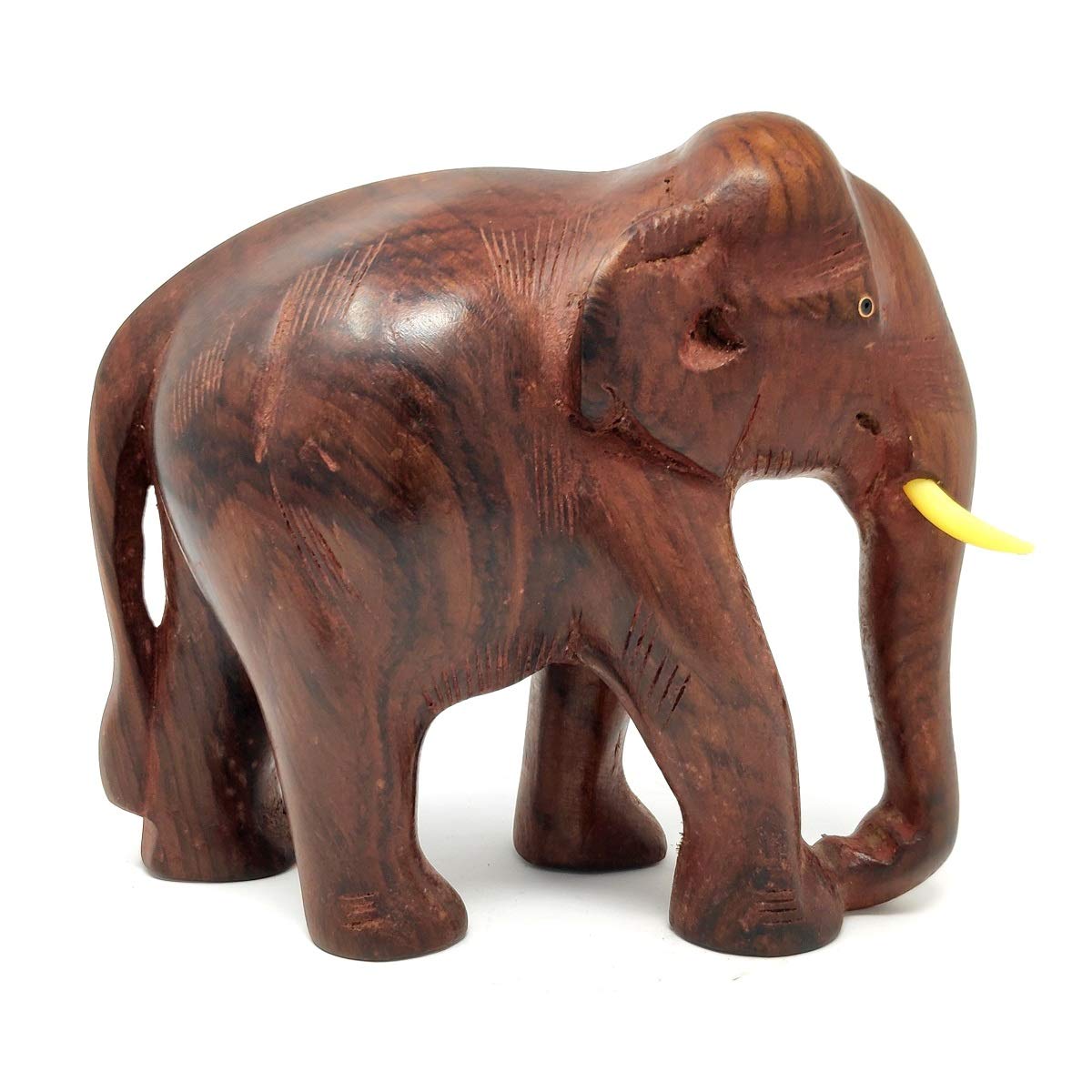The image depicts a highly detailed, handcrafted wooden elephant statue set against a solid white background. The elephant is carved from brown wood, showcasing intricate etchings and marks that suggest it is a hand-carved piece. The right side of the elephant is visible, including its right eye, trunk, and ear, which all feature elaborate detailing. The statue has a yellow tusk, possibly made of a different material, and its eye appears to have a metal inset, giving it a black and gold appearance. A notable feature is the lump on top of its head. The craftsmanship and novel detailing, including lines and notches, hint that this might be a souvenir from a safari in Africa. The statue’s trunk, which is attached to its front foot, and the etchings along its back and ear add to its rich texture and lifelike appearance.